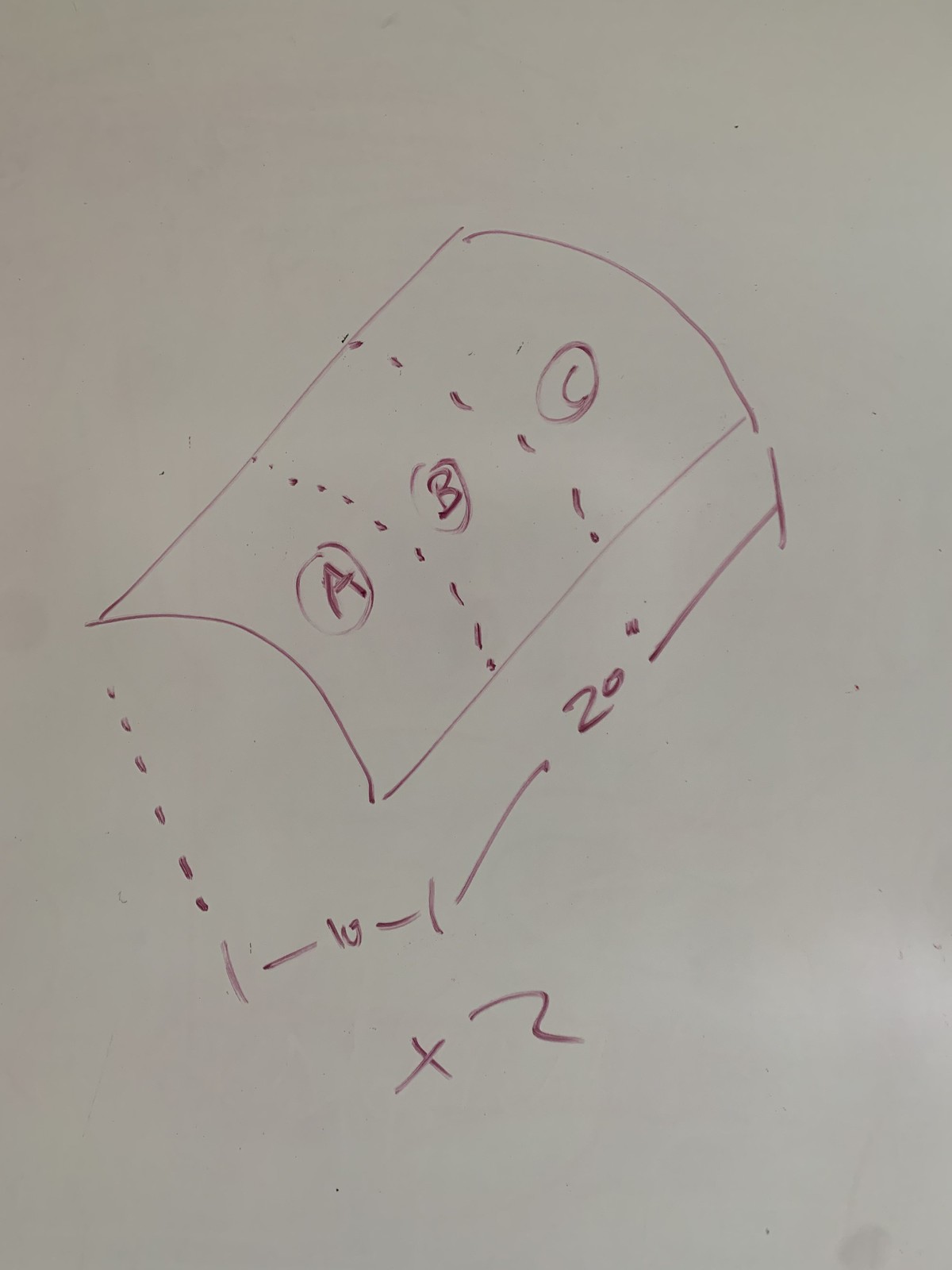This image, sketched on a gray piece of paper, features an arched, tunnel-like drawing that gives a three-dimensional illusion as if the paper itself is curving upward. The artist created a sense of depth by curving the sides of the arch. The drawing is segmented into three sections, labeled A, B, and C, with each section circled. The labeling appears to be done using a slightly faded magic marker, making the letters somewhat difficult to read.

Section A and B are separated by a series of small dots, while sections B and C are divided by larger, line-like dots. The dimensions are meticulously noted: along the side, a line indicates the measurement of 20 inches, marked by a double prime symbol (20″). Additional lines running down the side, which aren't visible under the arch, show measurements at intervals — 1 inch, 10 inches, and another 1 inch, with a notation of "times 2," reflecting the measurement of both sides of the arch combined.

Overall, the drawing showcases an intricate play with perspective, enhanced by the detailed and somewhat faded annotations.